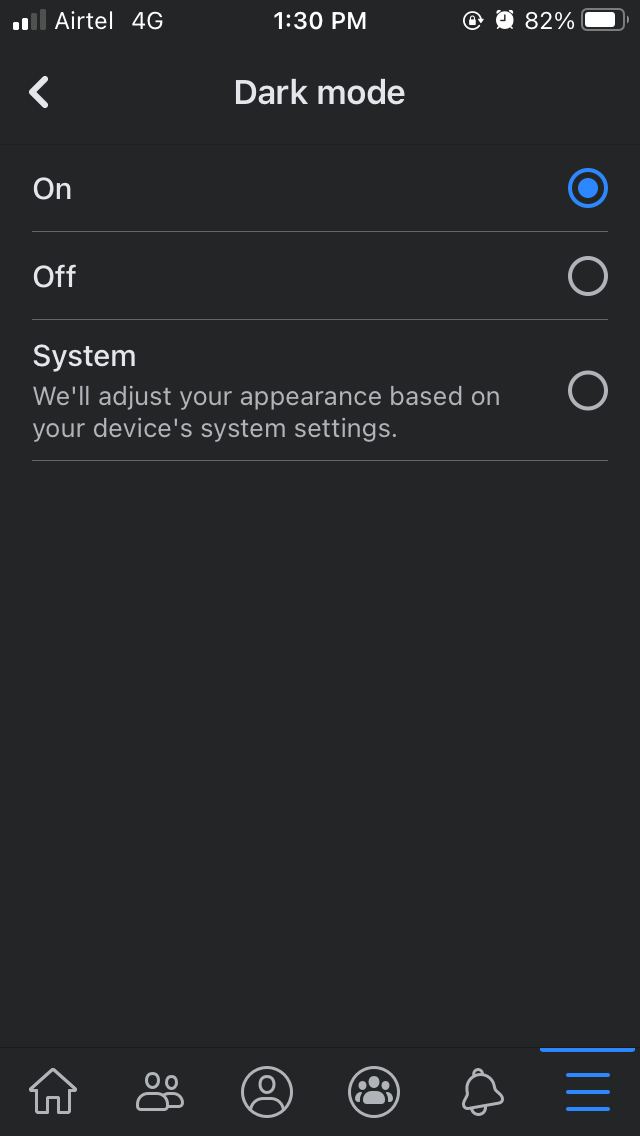This screenshot captures a smartphone interface in dark mode, where the background is black. In the top left corner, the network signal strength is indicated by two white and two gray bars, alongside the carrier name "Airtel" in white, which is misspelled as "A I R T E L." The 4G network indicator is placed next to it. At the center of the status bar, the time is displayed as "1:30 p.m."

On the right side of the status bar, an almost fully charged battery icon is shown with 82% indicated to its left, and an alarm clock icon is adjacent to it. Another element is a white circle with a black ring around it, bordered by another white ring.

Underneath the network details, there is a left-pointing greater than sign “>”. Directly beneath the time, "Dark mode" is written in bold white letters, followed by an "On" label on the left. On the right, a blue circle with a black border and a subsequent blue border is featured.

Below this, on the left side, there's a gray-bordered circle with a black interior and a horizontal gray line inside. The "System" label in white text appears slightly smaller, with a description: "We'll adjust your appearance based on your device's system settings."

Further down, there's empty space occupying about half of the screen until an inch from the bottom. Here, several icons are displayed in gray borders: a home icon, a people icon, and a profile icon, followed by a circle with three profile icons inside, and then a notification icon. On the right, three short blue horizontal lines are stacked, one above the other, with a longer blue line above them.

This detailed description comprehensively covers the visual elements and layout seen on the smartphone screen in dark mode.